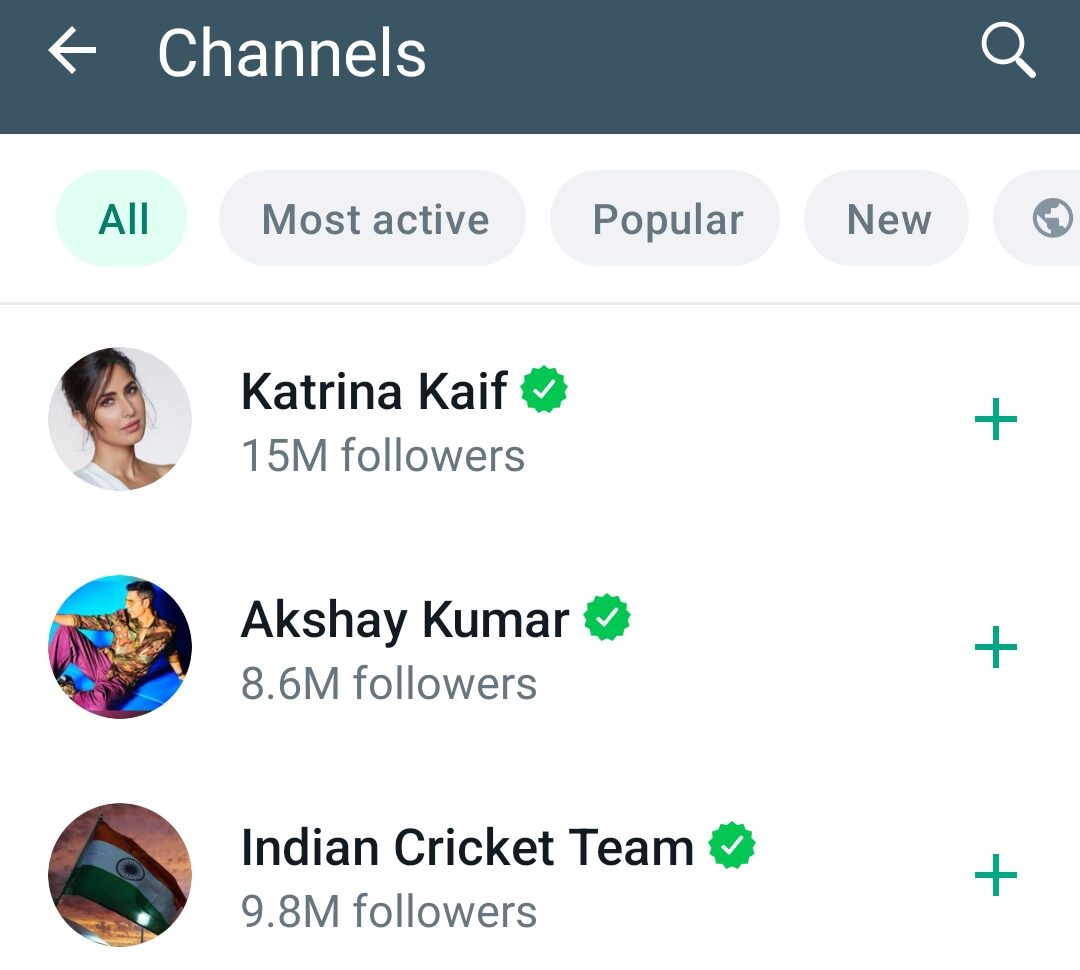This image is a screenshot from a mobile device, showcasing a user interface for managing channels. At the top of the page, a bluish-colored bar stretches horizontally across the screen, featuring a white back arrow on the upper left and the word "Channels" in white text towards the center. On the upper right corner of this bar, there is a search icon.

Directly beneath the blue bar, the screen has a white background. At the top of this white section, there are tabs for different categories, including "All" (which is highlighted in green as it is currently active), "Most Active," "Popular," and "New." A globe icon is situated to the right of the "New" tab. A light gray line separates these tabs from the content below.

The content area features a list of users and a cricket team, with detailed information for each. First, there is a photograph of Katrina Kaif, showing that she has 15 million followers along with a green plus symbol to follow her. Next, Akshay Kumar is listed with 8.6 million followers, accompanied by a similar green plus symbol for following. Lastly, the Indian cricket team is mentioned with 9.8 million followers, along with another green plus symbol to follow them. Each of these accounts is marked with a green checkmark, indicating their verified status.